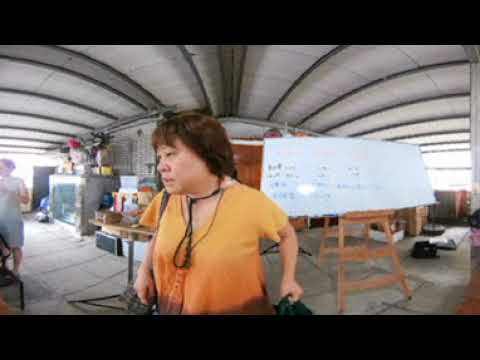In this detailed photograph, we see a woman dressed in a very light orange blouse, carrying a couple of bags and possibly rushing through the scene. She has medium-length turquoise hair and is wearing a black strap around her neck, with some beads that suggest a hint of religious significance, possibly Hindu. The setting appears to be an indoor facility that combines elements of an industrial and commercial space, somewhat resembling a warehouse. This is indicated by the presence of various items such as tables, workbenches, and what seem to be display kiosks or booths. 

In the background, there is a whiteboard with drawings or writings on it, contributing to an informal, workshop-like atmosphere. To her left, there is another woman, partially obscured, standing near a table with books, possibly involved in some sort of activity. The ceiling has an industrial, gray, and metal-like appearance, and other elements in the background include plants and potentially statues, adding a slightly eclectic feel to the environment. The image itself is framed with a black border at the top and bottom, adding to the overall composition.